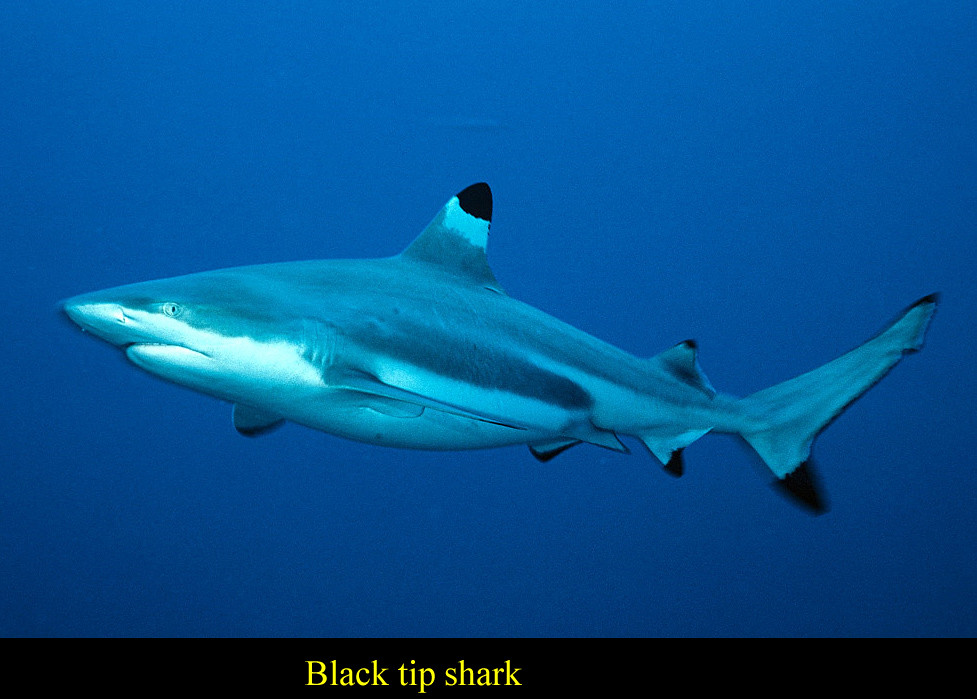The photograph is a clear, well-lit underwater scene showcasing a large shark prominently in the center, swimming against a vibrant blue backdrop. The shark, facing towards the left with its tail appearing slightly lower than its head, displays distinctive black tips on its dorsal fin, pectoral fins, and tail. Its body transitions from black-tipped fins to silvery hues and white edges, giving it a striking and detailed appearance. At the bottom of the rectangular image, a thick black banner extends across, housing the caption "Black Tip Shark" in bright yellow, simple font. This meticulously composed image, likely suitable for a science book or an aquarium display, captures the essence of the Black Tip Shark in its natural or displayed habitat.